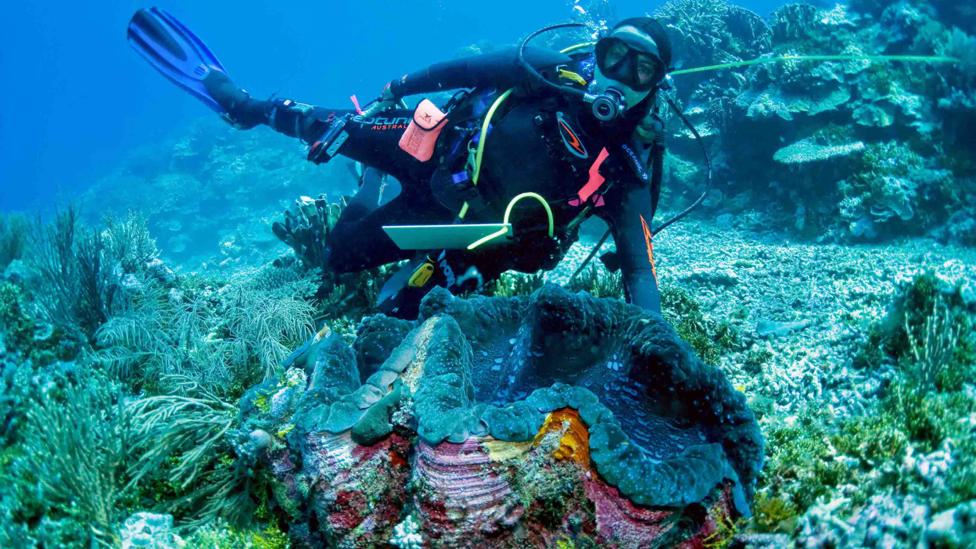This captivating underwater photograph portrays a scuba diver, possibly a woman, in full deep-sea diving gear, making it difficult to discern their gender. The diver, wearing a skin-tight, dark-colored suit with neon accents, occupies the nearly top center of the frame, slightly to the right, with their head almost touching the top edge of the image. The diver's head and hair are fully covered by the outfit, and they sport a face mask with a breathing apparatus. A black tube connects the mouthpiece to the oxygen source, with bubbles occasionally emanating from it.

The diver is oriented horizontally, with their right side closer to the camera. Their left leg is bent at the knee, adorned with a dark blue fin, adding dynamism to their posture. A pink pouch is attached to the diver’s hip, highlighting the otherwise monochromatic ensemble.

In the scene, the diver appears to be presenting a massive clam shell or coral structure, roughly half as large as the diver themselves. This remarkable object, with a bluish-green exterior and stunning pinkish hues within, adds intrigue and beauty to the composition.

The backdrop features the ocean floor adorned with multicolored coral and green plants, creating a vivid, textured landscape. While the upper left corner fades into the deep blue void of the sea, the rest of the image is rich with the aquatic life and rocky areas that frame this underwater exploration. The interplay of light and color, with shades of teal and deeper blue, underscores the serene, natural beauty of the ocean depths.